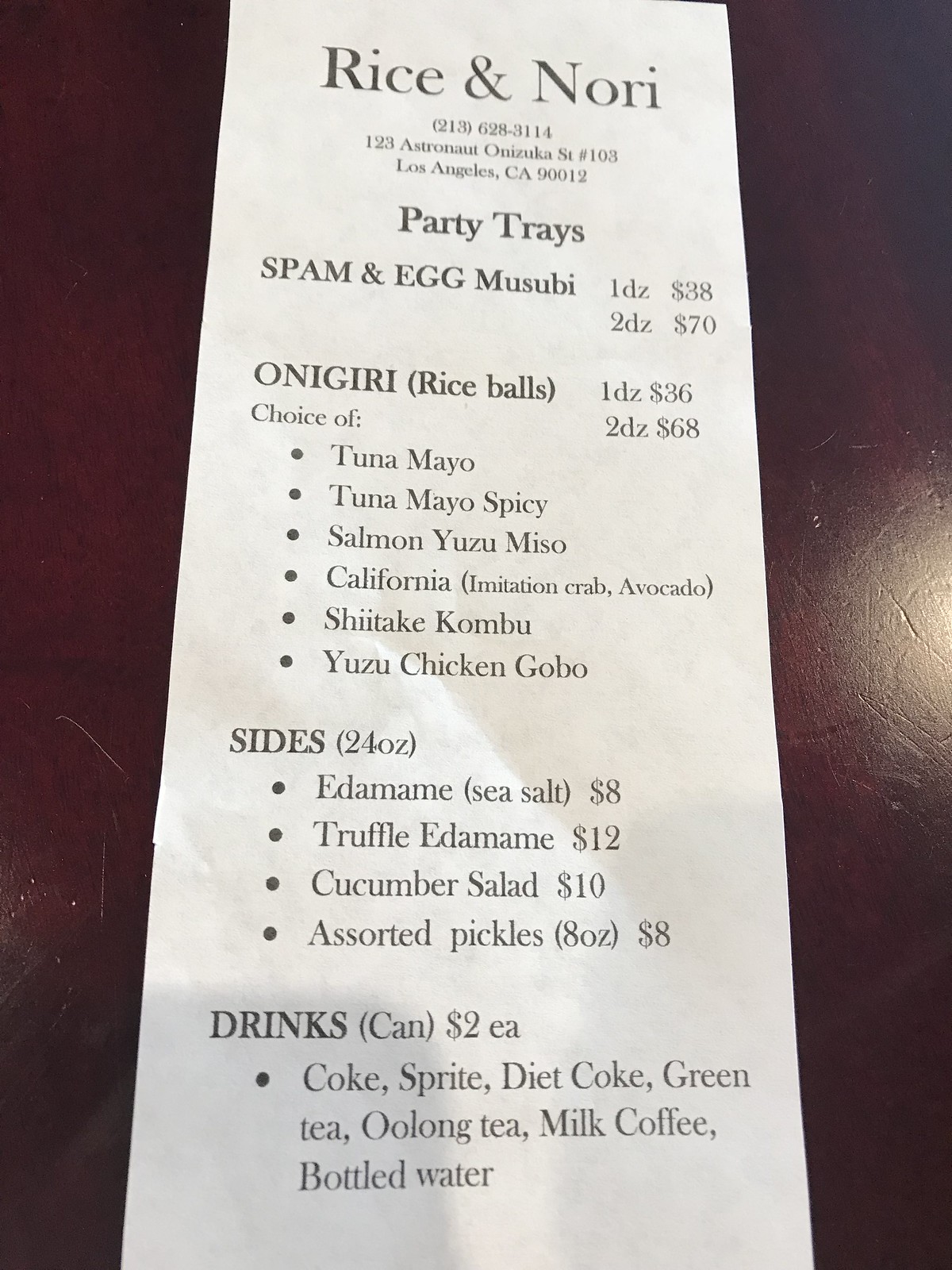This image features a detailed photo of a receipt from "Rice and Nori," a restaurant located at 213-628-3114, 123 Astronaut Azuco Street, Suite 103, Los Angeles, California. At the center of the receipt in bold, it lists a party tray that includes "Spam and Egg Musubi." Below this, a variety of Onigiri (rice balls) options are detailed, featuring different fillings: Tuna Mayo, Spicy Tuna Mayo, Salmon Yuzo Miso, California (Imitation Crab and Avocado), Shiitake, Kombu, Yuzo, and Chicken Gobo.

Additionally, the receipt lists several sides available in 24oz portions, including Edamame with Sea Salt priced at $8, Truffle Edamame, Cucumber Salad, and Assorted Pickles.

For beverages, the receipt offers a range of drinks including Coke, Sprite, Diet Coke, Green Tea, Oolong Tea, Milk, Coffee, and Bottled Water.